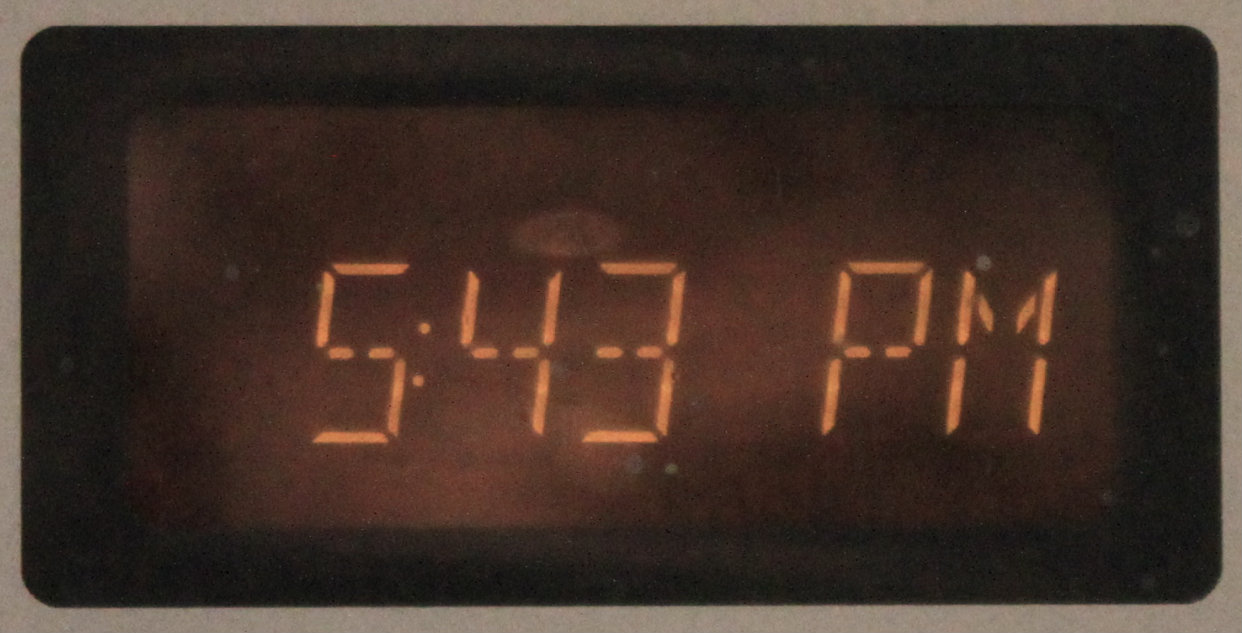A grainy photograph showcases a standard digital alarm clock positioned centrally against a plain beige background. The clock features a sleek black frame surrounding the display. The time, shown in a retro 1980s digital font, reads 5:43 PM with the colon between the hours and minutes clearly visible. The digits are illuminated in a reddish-orange hue, adding a vintage feel to the image. Despite the graininess of the picture, the digital display is sharp and free of pixel burn or any distortions, making the time easily legible.